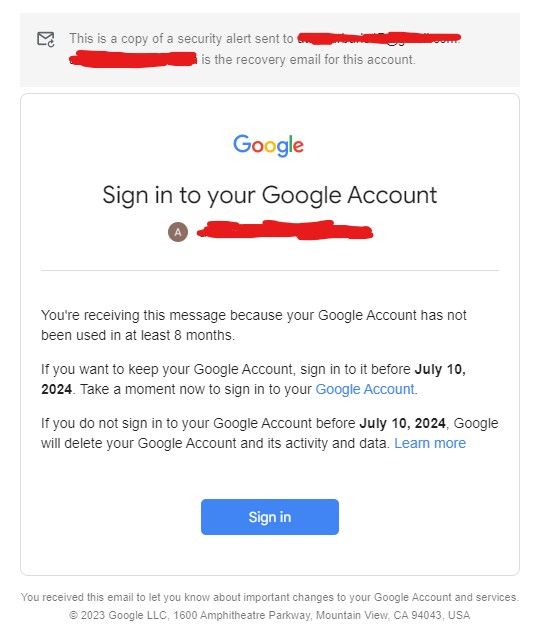The image displays a stylized screenshot of a security alert email from Google regarding account inactivity. At the top, there’s a light gray banner featuring a dark gray envelope icon on the left, with a refresh button on the bottom right corner of the envelope. This banner contains red strike-through text, "This is a copy of a security alert sent to you." Below it, uncrossed, reads, "is the recovery email for this account."

Transitioning into the main body, there’s a white section bordered lightly in gray with rounded corners. Centered at the top is the Google logo. Beneath it, in bold black text, it states, "Sign in to your Google Account." To the left, a user icon appears as a brown circle with a white capital "A." The username next to it is redacted. A gray dividing line separates this header from the message content, which explains in black sans-serif text that the user’s Google account has been inactive for at least eight months. The crucial information is bolded: "sign into it before July 10, 2024," with the clickable "Google account" link in blue. It continues detailing the consequences of inaction, emphasizing that the account and its associated data will be deleted if not accessed by the specified date. The term "Learn more" is also in blue, indicating a hyperlink.

At the bottom center of the white area, there's a blue rectangular button with rounded corners stating "Sign in" in white text. The footer in small gray text alerts the reader about vital changes to their Google account and services, followed by the legal copyright information: "Copyright 2023 Google LLC, 1600 Amphitheater Parkway, Mountain View, CA 94043 USA."

This descriptive caption provides a comprehensive overview of the image, detailing the layout and contents of the email screenshot.